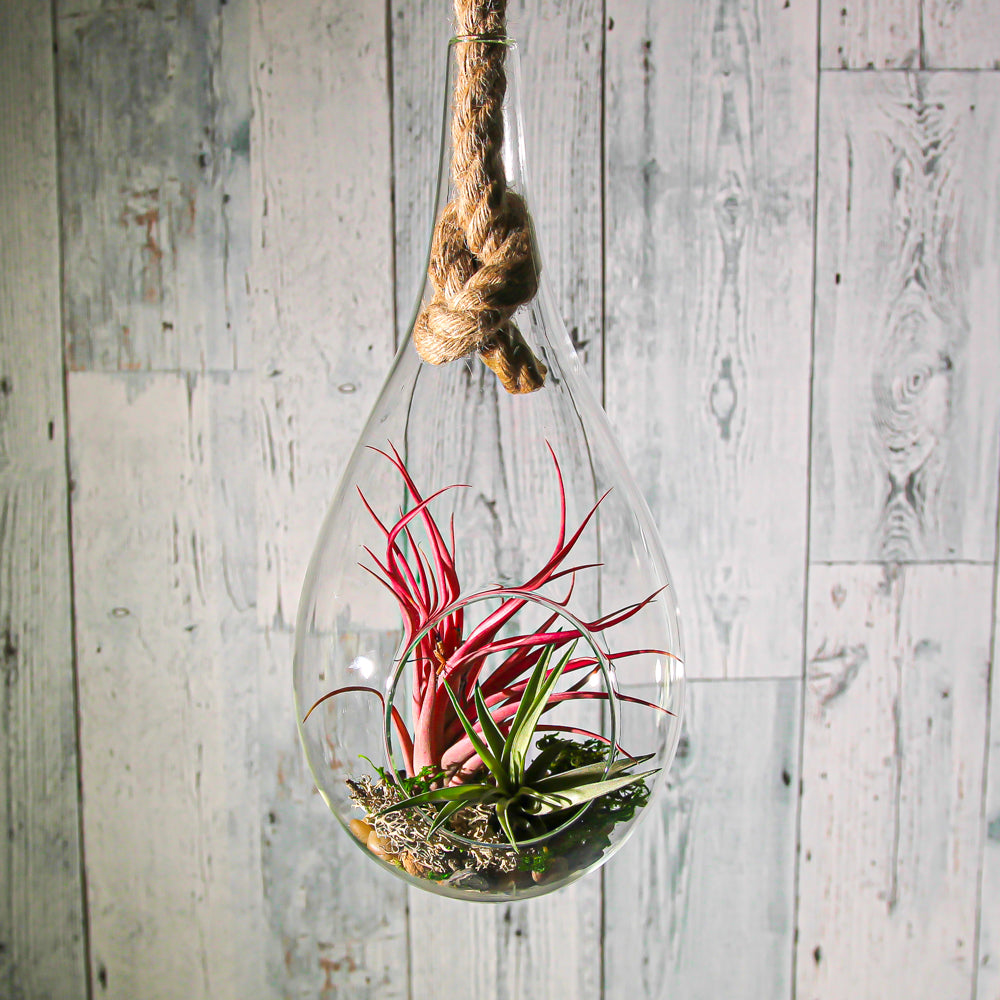This photograph showcases a teardrop-shaped glass terrarium orb, approximately palm-sized, elegantly suspended by a sturdy piece of nautical, jute rope tied into a knot at the terrarium's top. The backdrop features wide, weathered white wood planks with a shabby chic appeal. Inside the clear glass terrarium, which has a front opening for easy plant maintenance, lies a picturesque arrangement of small rocks and soft moss at the base. Nestled in this bed are two distinct plants: a green spider plant with a spiny appearance, and a striking red succulent resembling a spider plant but differentiated by its vibrant color. The glass orb, hanging serenely, commands attention against the rustic yet charming wooden background.